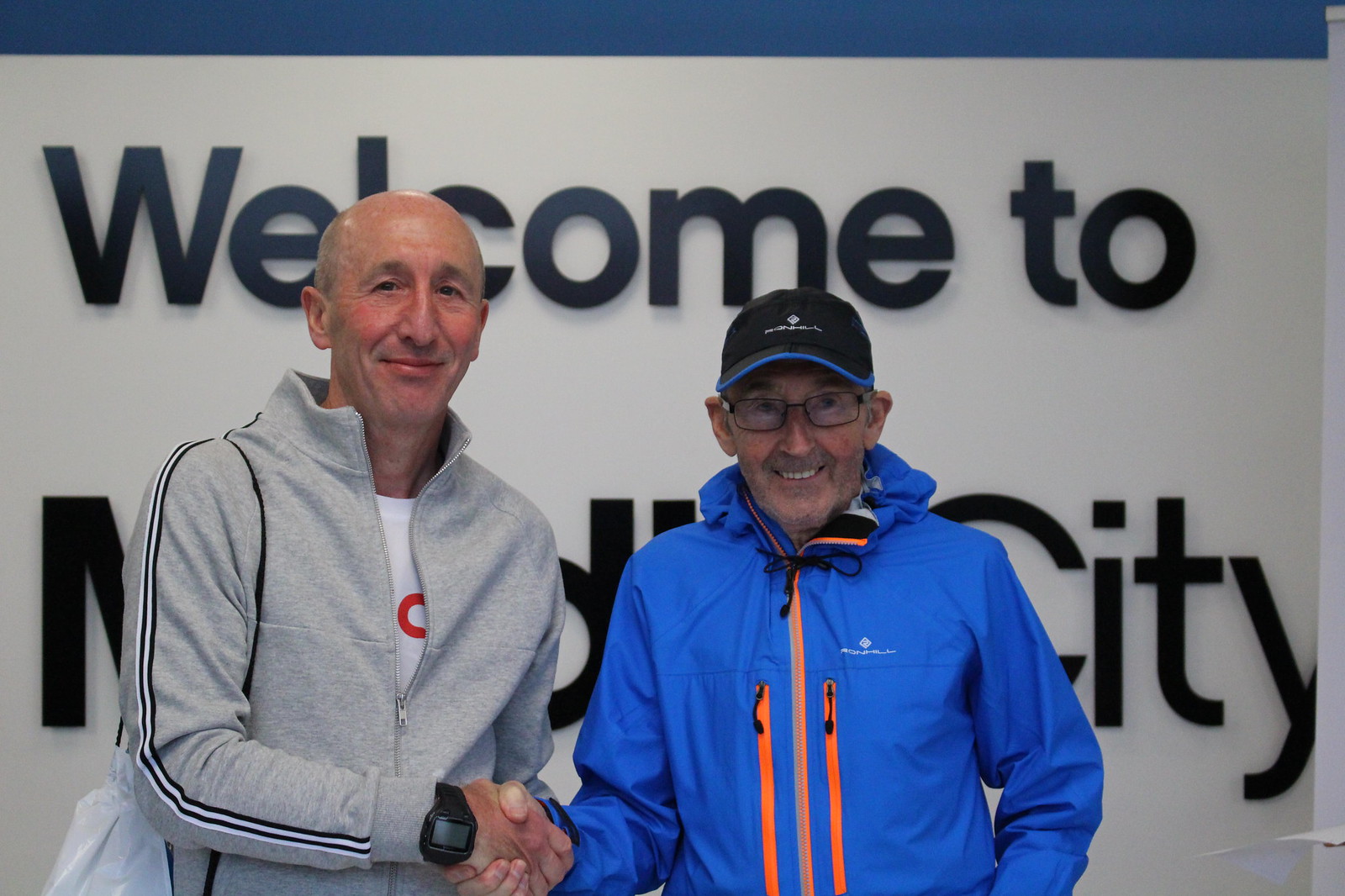In this detailed image, we see two men shaking hands in front of a decorated wall with three-dimensional letters that spell out "Welcome to [partially obscured] City" on a white background. Both men are facing the camera and radiate friendly expressions. 

The man on the left is taller, bald, and has no facial hair. He is wearing a gray workout sweatshirt that is partially unzipped, revealing a white t-shirt underneath with some red text. His left wrist sports a thick black watch, and he carries a white bag with a black strap slung over his right shoulder. 

The man on the right wears a bright royal blue windbreaker jacket with a hood and distinctive pinkish-orange zippers. His black baseball cap features a blue rim and white writing. He has rectangular glasses, a scruffy beard, and a warm smile. The detailed contrast between the men’s attire and the partially revealed greeting behind them adds a welcoming and vibrant aura to the scene.